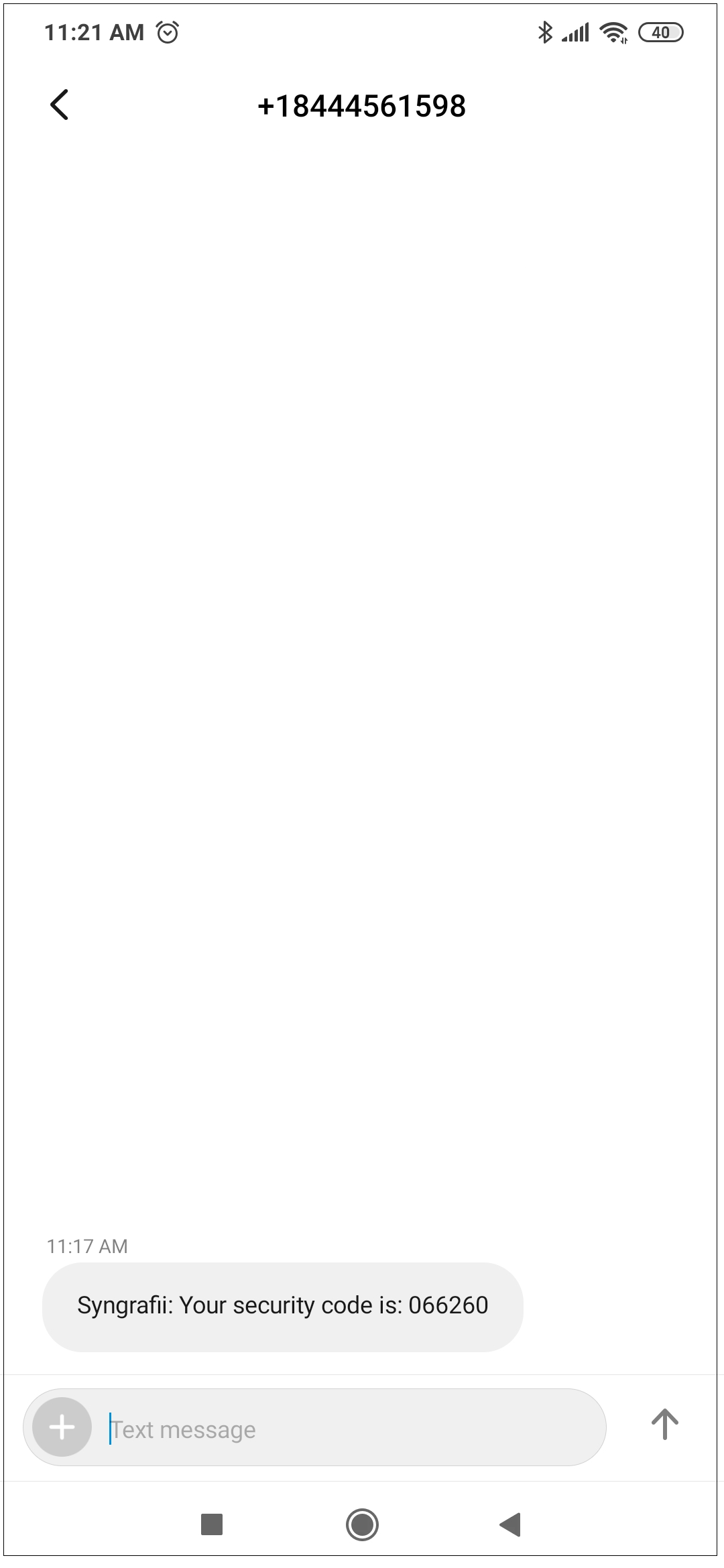This image is set against a white background framed by a thin gray line, forming a vertical rectangle. At the top center, the text "11:21 a.m." appears in black, accompanied by an alarm clock icon. To the right of this, a sequence of symbols conveys various statuses, including a Bluetooth icon, a Wi-Fi signal, a cellphone signal indicator, and a battery icon displaying "40." 

Below this, at the center of the top section, bold black text reads "+18444561598." Further down, at the bottom of the image, the time "11:17 a.m." is displayed with "A.M." in capital letters. 

There is also a lengthy oval-shaped text bubble containing the message: "Syngraphii: Your security code is: 066260," where "Syngraphii" is spelled with capital letters "S-Y-N-G-R-A-F-I-I" followed by colons. Below this, another arrow points upwards, indicating a subsequent option for another text message.